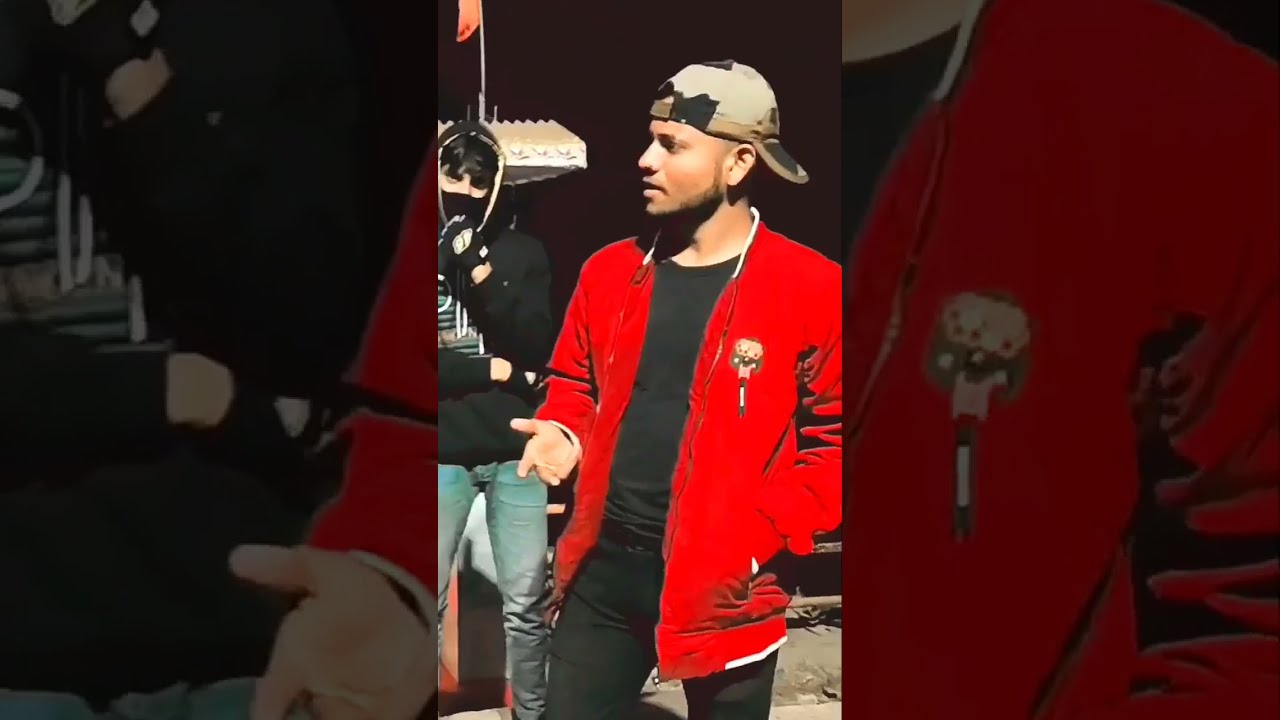The image, seemingly captured outdoors, is a composite of three panels featuring two individuals and their details. In the central panel, there's a young man with brown skin, dressed in a backward beige cap, a black shirt, and black jeans. He sports a red hoodie with an unzipped front, showcasing a small bear emblem. His right hand extends outward, while his left hand rests in his pocket. He faces left, engaging with someone out of the frame. In the background, another man wears a black hoodie, complemented by a black mask that conceals his face. He adopts a direct stance towards the camera, with his right hand across his stomach and left hand raised to his mouth, paired with blue jeans. The left panel zooms in on the red hoodie and the man's hand from the central scene, while the right panel provides a close-up of the same red hoodie, emphasizing its distinct bear logo. The color palette across the image includes black, white, blue, red, gray, brown, and orange, creating a cohesive yet detailed screenshot potentially taken from a mobile device, possibly Instagram or TikTok.